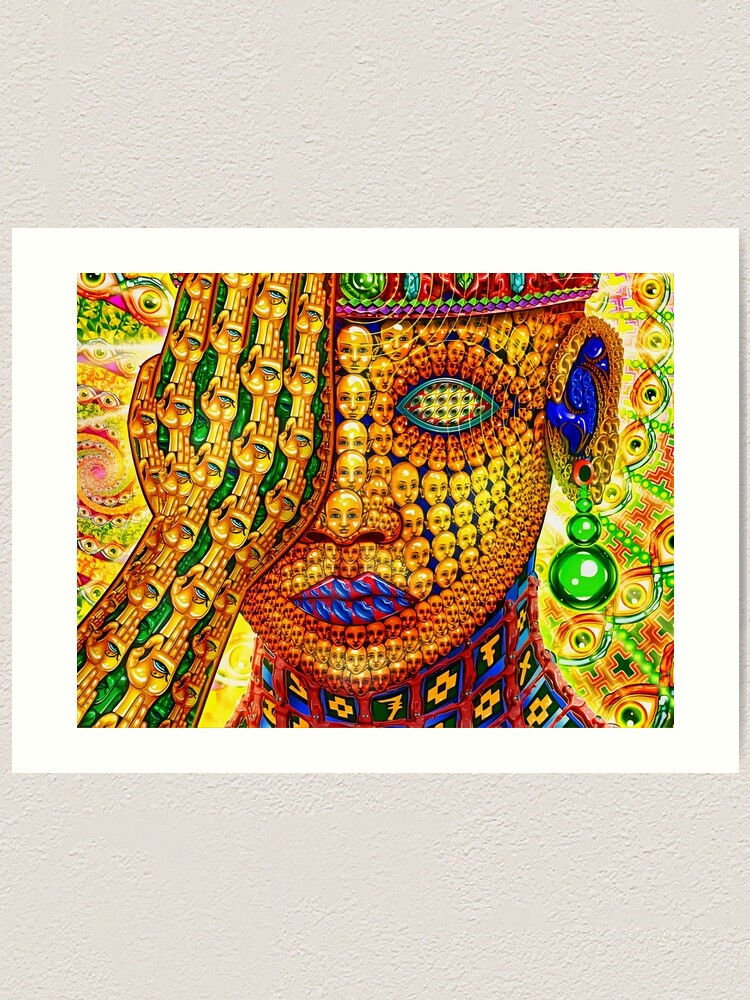The rectangular image, measuring approximately five inches high and four inches wide, features a striking psychedelic artwork. In the center of a white stucco background, a smaller horizontal rectangle frames the main subject — a surreal depiction of a head and right hand. The head, composed of tiny golden faces, exudes a somewhat eerie vibe while the golden hand, interspersed with smaller green hands, covers the right eye. The golden hand is adorned with delicate blue eyes that seem to stare directly at the viewer. The person's face is further detailed with sections made of smaller skulls and red and blue lips, enhancing the intricate and bizarre aesthetic. The neck, colored in reds and adorned with blue and green squares with numbers, extends downwards, bordered by strands resembling DNA helixes. These strands incorporate various colors including yellows, greens, blues, and oranges, with eyeballs and crosses interspersed amongst them. Surrounding the main figure, a swirling spiral and additional psychedelic striations add to the overall otherworldly and complex composition of the image.